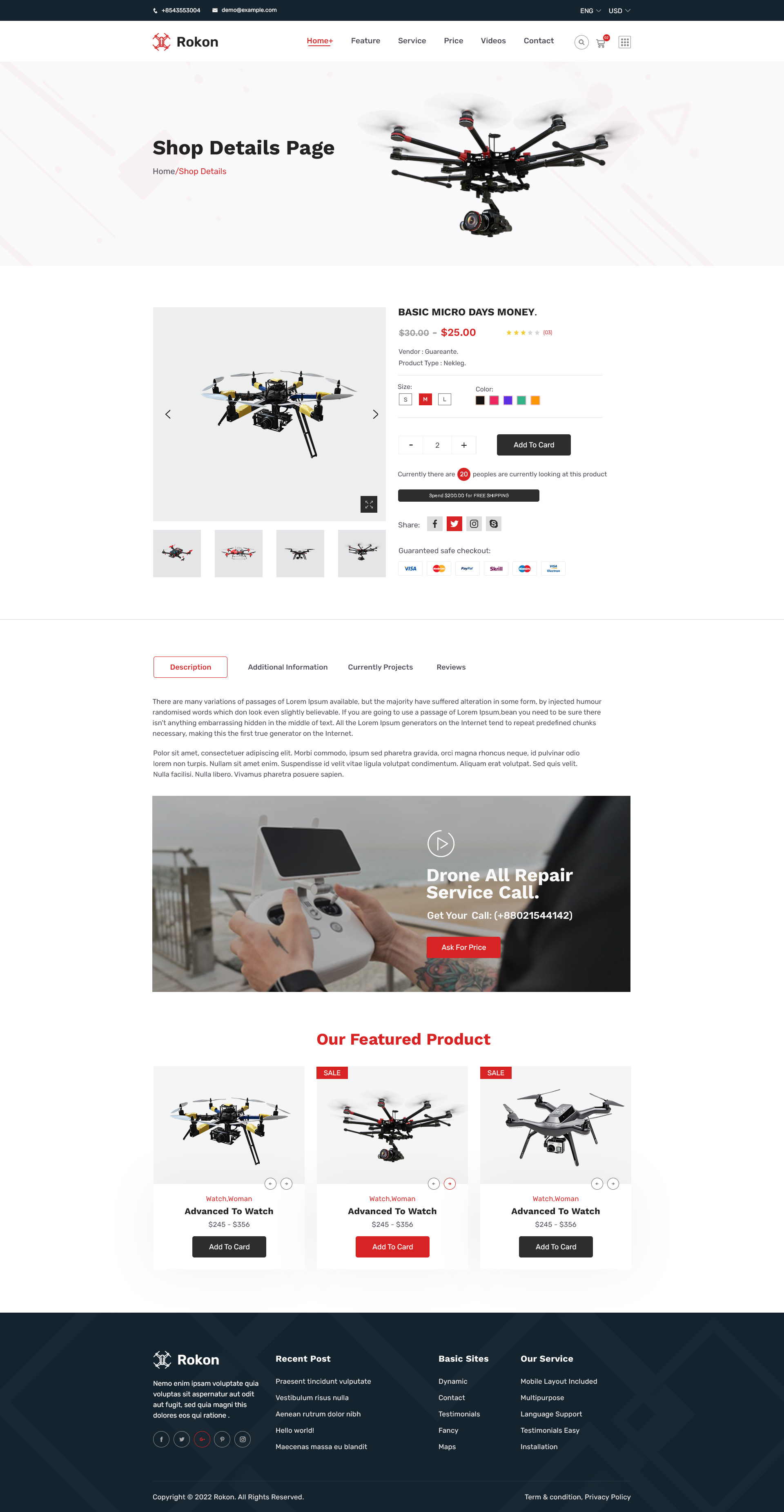**Detailed Caption:**

The image depicts a comprehensive screenshot of a drone-related webpage, presumably from a site called "Roken" (though the logo and name are somewhat small and unclear). The layout extends the entire length of the screen. At the very top is a navigation menu, followed by a prominent, large image of a drone with the text "Shop Details Page" underneath. Below that is a smaller drone image accompanied by several other thumbnails arranged for horizontal scrolling.

To the right of the images, detailed specifications of the highlighted drone are displayed, including the model name, price, and available color options. Proceeding further down, there is an informational section divided into four sub-menus or tabs, one of which is highlighted but illegible. The sections might include categories such as "Products" and "How to Operate," followed by descriptive paragraphs.

Below the text, there's an image with the caption “Drone All Repair Service Call” next to a conspicuous red button intended for initiating a service call. Further down is a section titled “Our Featured Product,” showcasing three smaller drone images, likely emphasizing top products.

The bottom of the webpage features a typical footer section containing various links to social media profiles, as well as navigational links to different sections of the site.